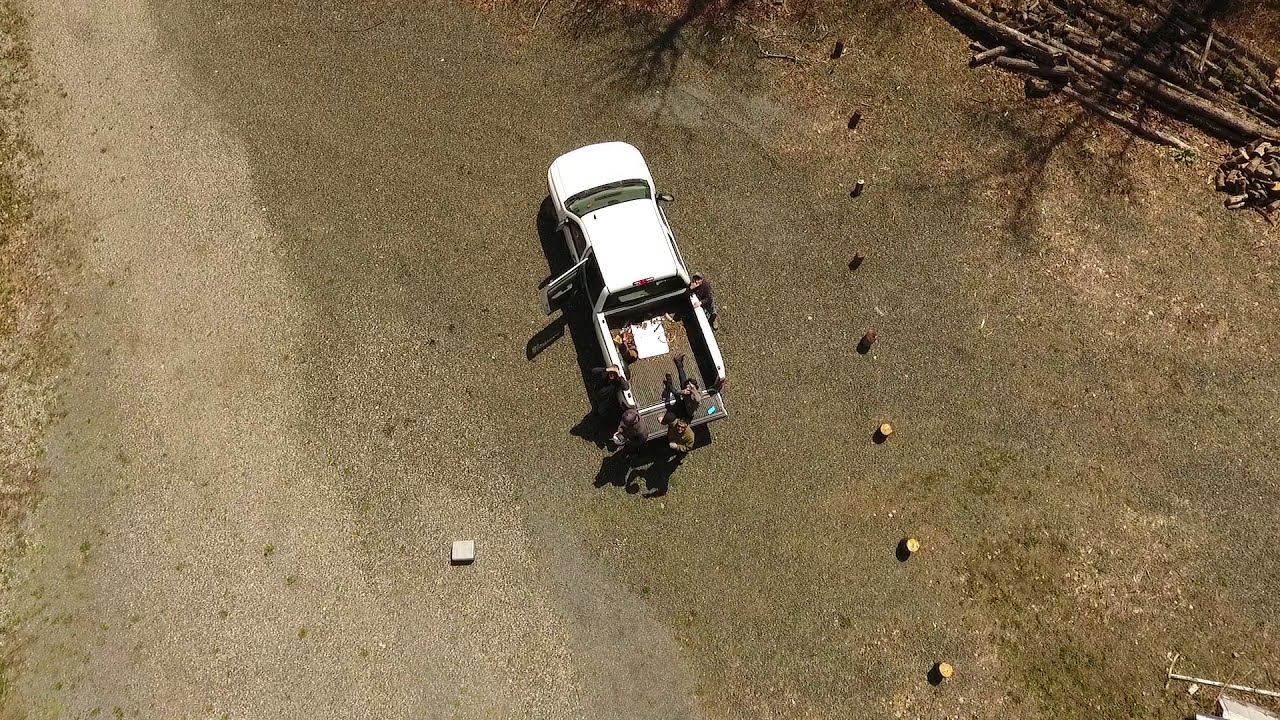This aerial photograph, likely taken from a drone, shows a top-down view of a white pickup truck centered in the frame. The truck is oriented with its front facing towards the top of the image and its driver's side door open. The bed is empty with the tailgate down. Four or five people are gathered around the truck, some sitting on the open tailgate, and others standing nearby, looking up at the drone. The scene is set on a flat, nondescript dirt ground with hints of brown and green, possibly suggesting a forest trail. In the upper right corner, there are some twigs or fallen tree branches. Along the right side of the truck, small wooden posts are arranged vertically, perhaps forming a barrier or demarcating a path.